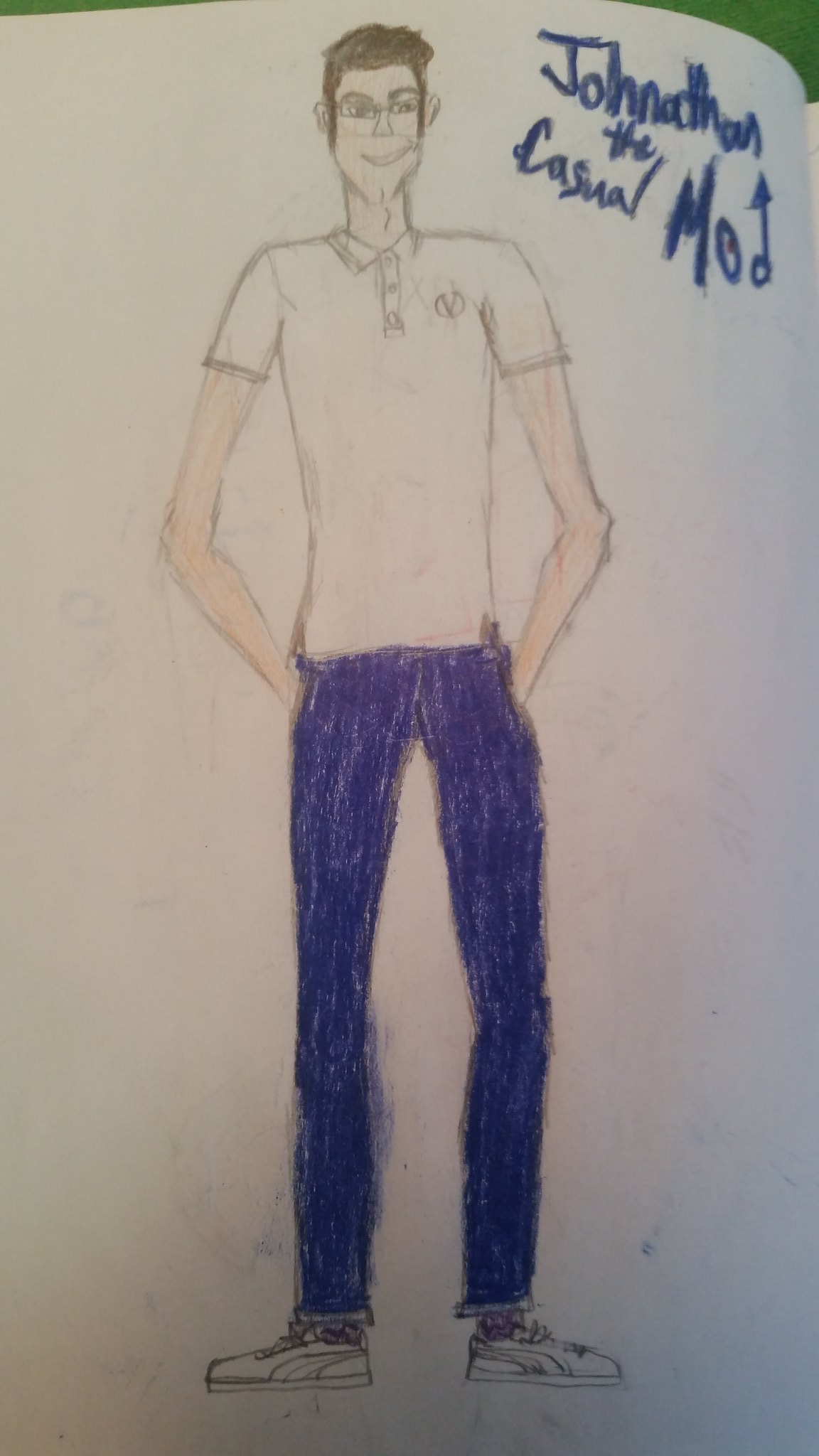This detailed drawing, done on white sketchbook paper placed on a dark green desk, features a young man with brown hair and peach-colored skin. The man, depicted with long sideburns, is smiling subtly. He wears a short-sleeved white polo shirt, untucked, with a logo resembling an upside-down 'A' or a fortune cookie on the chest. His dark blue pants are paired with white tennis shoes that resemble Puma sneakers. His hands are casually tucked into his pockets. 

In the upper right corner of the sketch, written in dark blue either crayon or pencil, is the name "Jonathan" followed by the text "The Casual Mod." "Mod" is uniquely styled with a capital "M" inside a circle and a "D" shaped line with an arrow at the top. The drawing's background includes intricate details of the sketchbook's pages with hints of other sketches faintly visible on the reverse side.